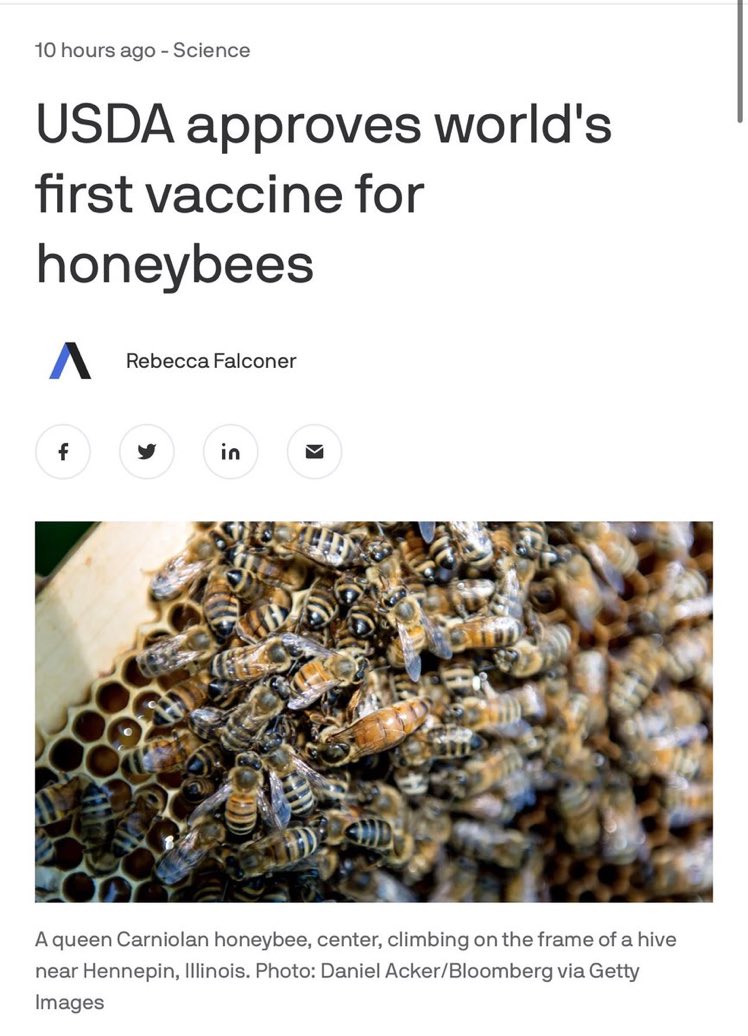The screenshot shows a news article from a feed, posted 10 hours ago under the category "Science". The main headline reads, "USDA Approves World's First Vaccine for Honeybees," authored by Rebecca Falconer. The article offers four ways to contact Rebecca, represented by icons for Facebook, Twitter, Indeed, and email.

A large photograph accompanies the article, depicting bees within a man-made hive. In the upper left-hand corner of the image, a small piece of wood is visible. The photograph specifically features a Queen Carniolan honeybee climbing on the frame of the hive near Hennepin, Illinois. This image was captured by Daniel Acker and is credited to Bloomberg via Getty Images.